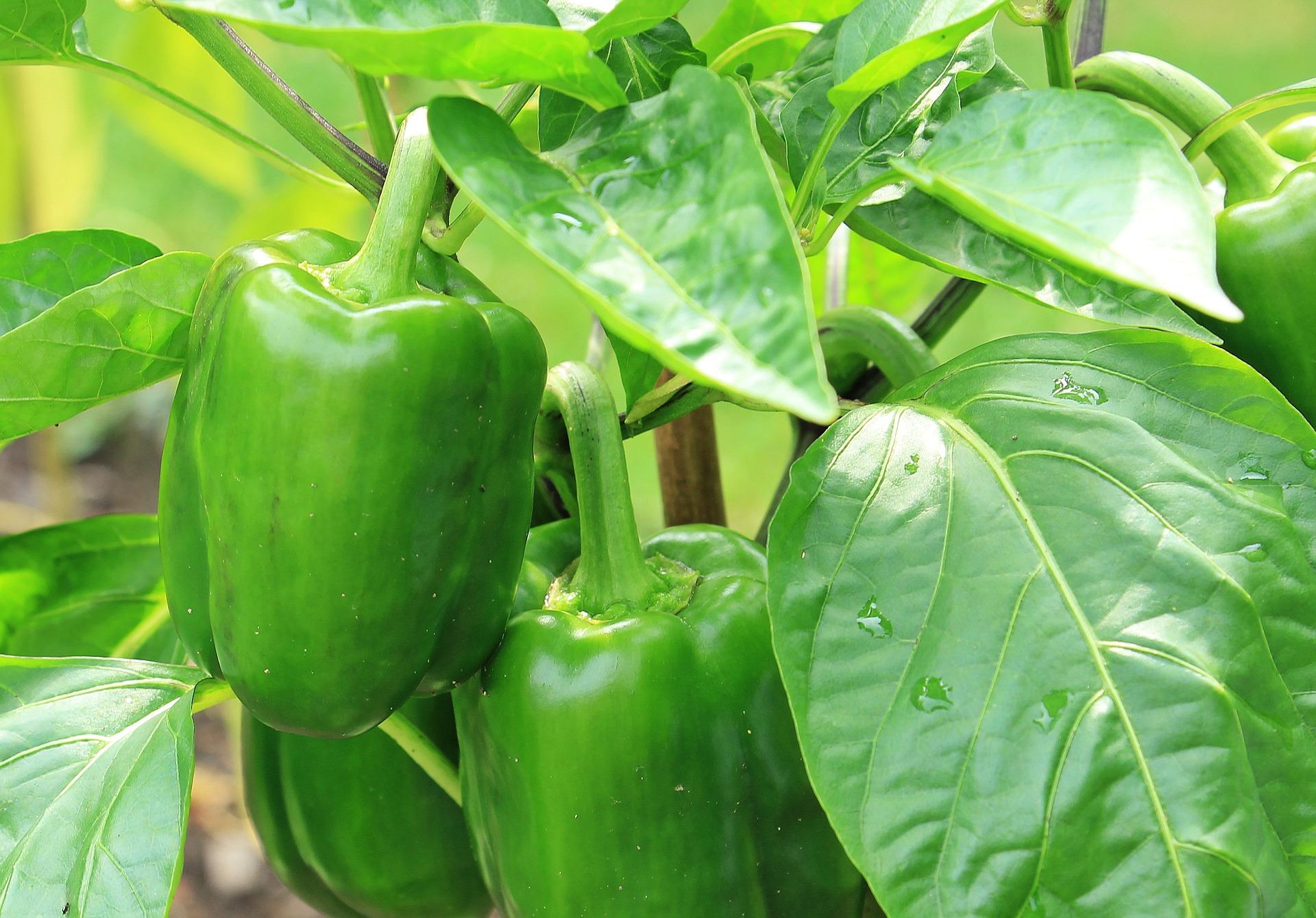This close-up image captures a vibrant green pepper plant with several bell peppers in various stages of growth. On the left side, two prominent, sizeable green bell peppers hang from the plant, one slightly above the other. To the right, the edge of another pepper is visible, partially out of frame. In the background, the blurred green hues suggest more foliage, possibly other plants. The plant's large leaves, some of which are even larger than the peppers themselves, dominate the frame, particularly noted in the lower right corner where a water-droplet-speckled leaf suggests recent watering or rain. Additionally, a brown stem is noticeable in the background, possibly part of the plant's structure. The image shows no visible sunlight or ground, focusing entirely on the thriving pepper-laden plant.